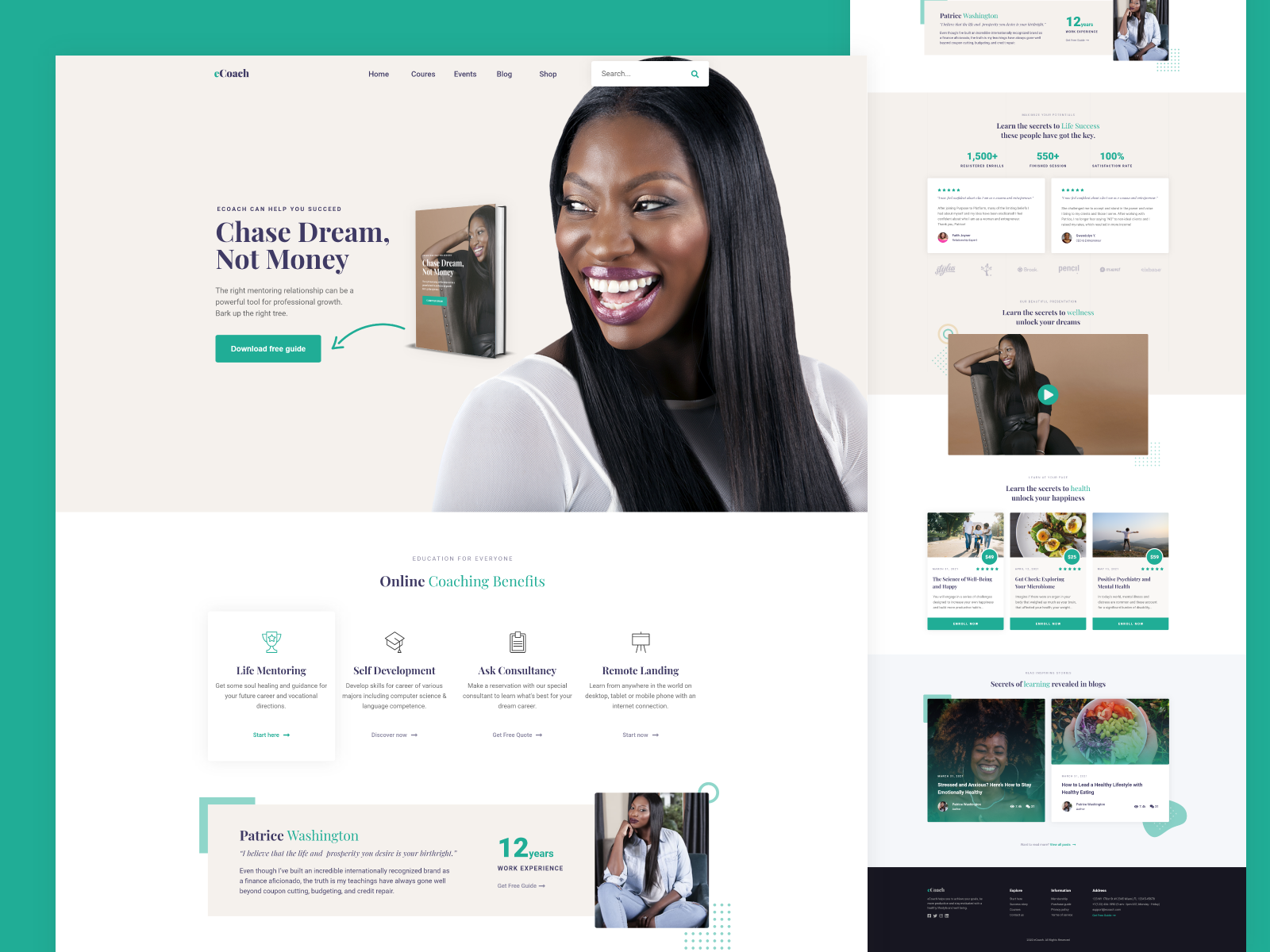Detailed Description of the Image:

The image is a detailed screenshot of a website portfolio with a teal green background, displayed in two distinct panels. The panel on the left showcases the upper section of a website, offering a closer view of the site's initial impression. The website logo in the upper left corner reads "Coach" or "Couch." The top section features a navigation bar with several options and a prominent search bar.

Central to the left panel is an engaging image of a woman smiling and looking off to the left, holding a book that appears to feature the same woman on the cover. The headline accompanying this image proclaims, "Chase Dreams, Not Money," along with a clickable link that likely reads "Download Free Guide."

Below this main section, bullet points highlight the benefits of online coaching, including Life Mentoring, Self-Development, Ask Consultancy, and Remote Lending. Further down, a brief bio introduces Patrice Washington, noting her 12 years of work experience.

The right-side panel continues from the main website view, displaying the content that follows as one would scroll down the page. It includes a thumbnail for a video, additional textual content, and potential blog articles. The vertical flow concludes at the footer, which contains standardized footer links commonly found on websites.

This comprehensive layout effectively presents an overall view and specific details of the website, emphasizing its emphasis on coaching and self-development.